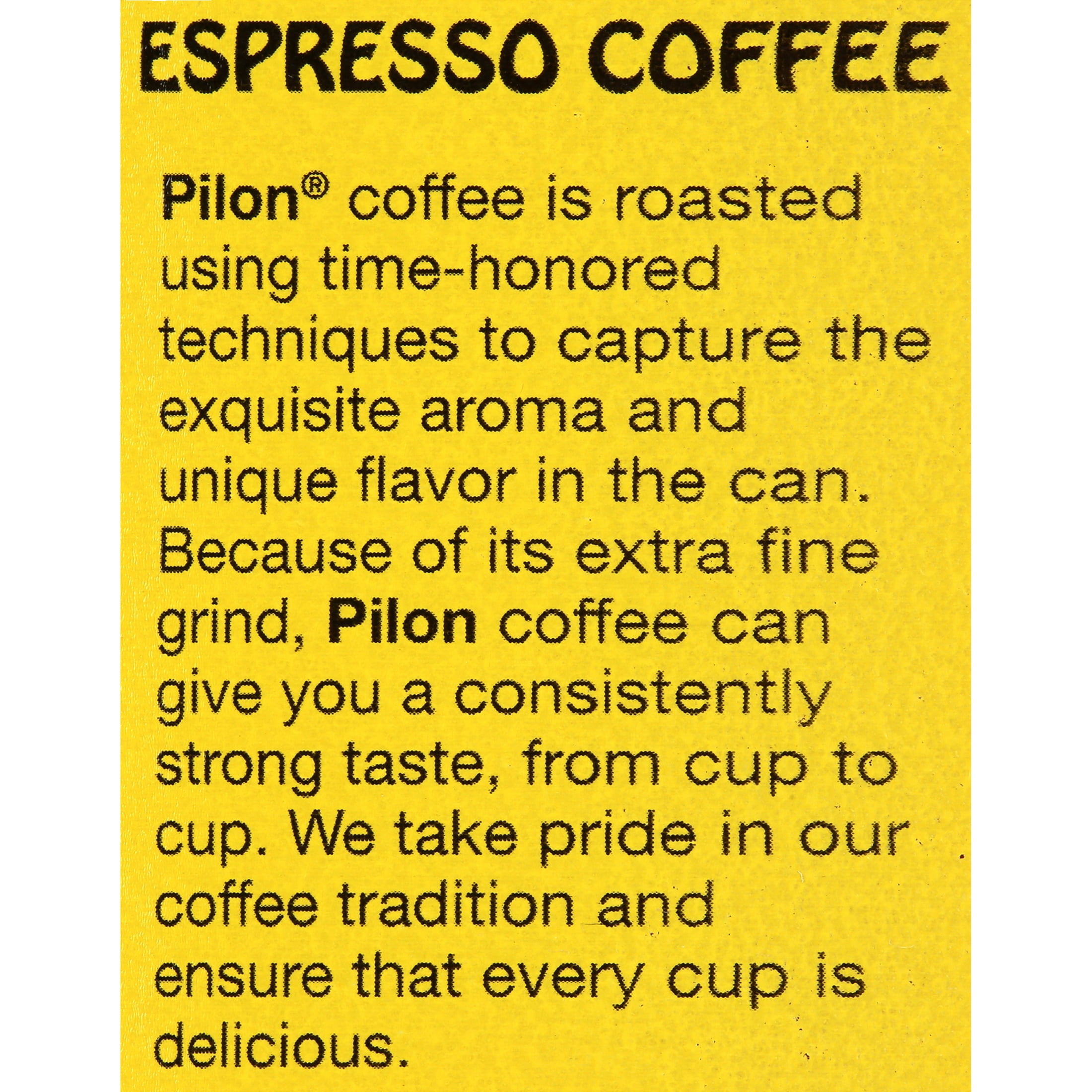This image is a graphic with a yellow background featuring prominently bold black text. At the top, "Espresso Coffee" is displayed in a large, bold font. Below, the text discusses Pilon coffee, starting with "Pilon" in bold with a registered trademark symbol. The detailed description follows, stating that "Pilon coffee is roasted using time-honored techniques to capture the exquisite aroma and unique flavor in the can. Because of its extra fine grind, Pilon coffee can give you a consistently strong taste from cup to cup. We take pride in our coffee tradition and ensure that every cup is delicious." The font used is reminiscent of a retro or basic, possibly Times New Roman style, which reinforces the straightforward and nostalgic design of the advertisement.